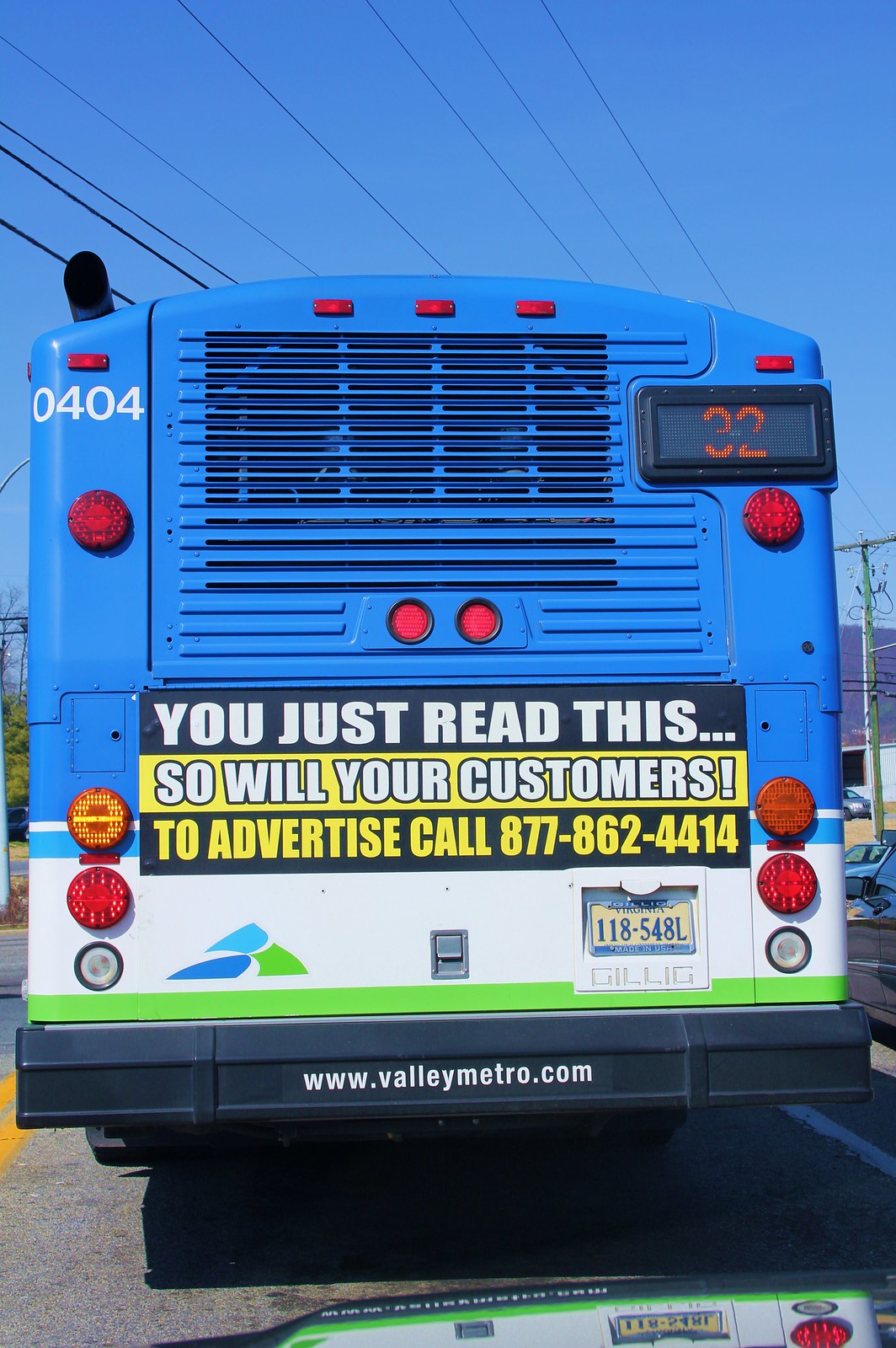This detailed photograph captures the back of a blue and white city bus driving on a street during the daytime. Dominating the image, the bus is framed against a clear blue sky adorned with power lines. At the top right corner of the bus, a digital sign glows with the number "32" in an orange-red light. Adjacent to it, another number "0404" is displayed in white. Centrally placed on the bus is an advertisement banner with the text: "You just read this, so will your customers. To advertise, call 877-862-4414." Directly below this banner is the license plate marked "Virginia 118548L." Beneath the license plate, a green stripe accentuates the otherwise blue and white bus. At the very bottom on the bumper, the website "www.valleymetro.com" is clearly visible. The setup and style of the photo emphasize an urban setting captured in a vertical rectangle, showcasing a clearly detailed city bus amid the vivid, daytime environment.